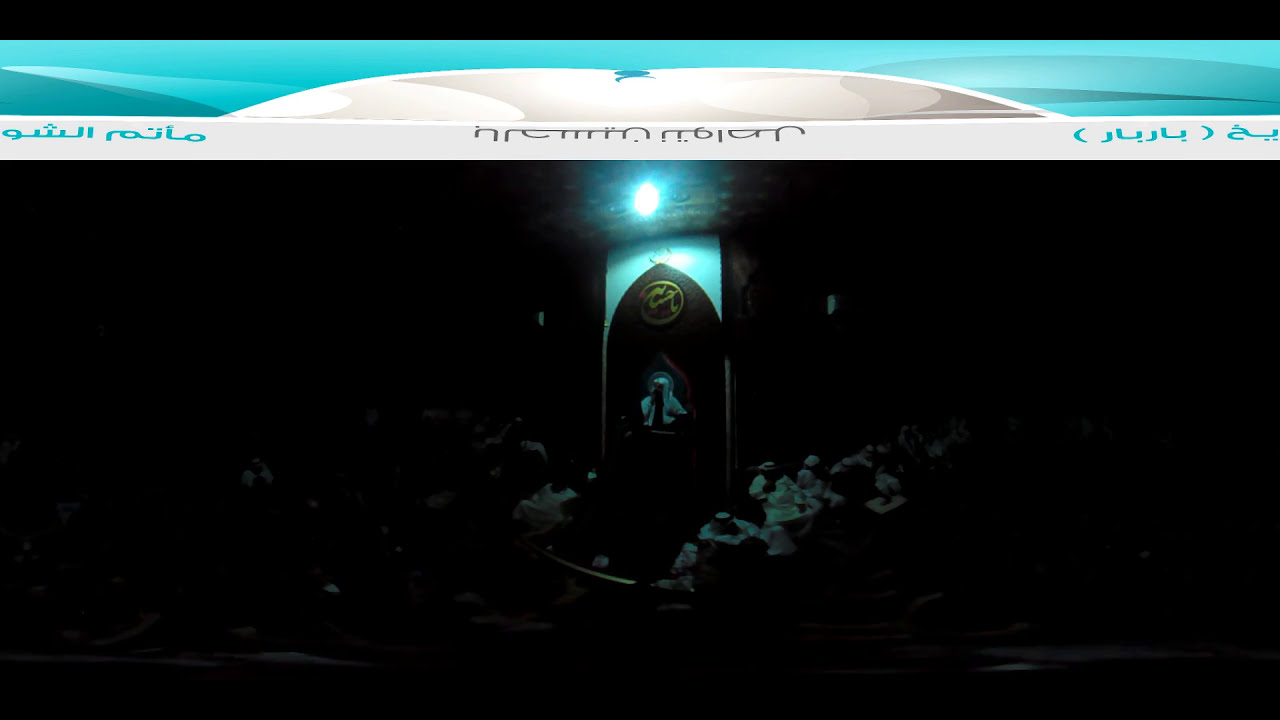The image depicts a very dimly lit indoor scene. Centered in the frame is a person who appears to be facing outward, possibly standing on a stage or a raised platform. Barely visible, this individual seems to be holding a microphone, suggesting they might be performing. Surrounding them, other individuals are faintly discernible, predominantly due to the light reflecting off their white clothing, forming a semicircle as they focus on the stage.

Taking prominence in the backdrop is a black arch structure with a light blue rectangle behind it. Within the arch, a raised or embossed image is visible, crowned by a small yellow circle emblazoned with an emblem. Above this arch, recessed lighting casts a blue haze across the ceiling, adding to the obscure ambiance.

Spanning the top of the image is a light blue banner adorned with a semicircular white logo and what appears to be Arabic writing, flanked by blue text on either side and black text in the middle. Another blue and white banner, displaying decorative lines, runs parallel above the first, both bordered by thin black strips at the top and bottom. The information collectively presents a dark, enigmatic venue, potentially a Middle Eastern-themed event or performance.